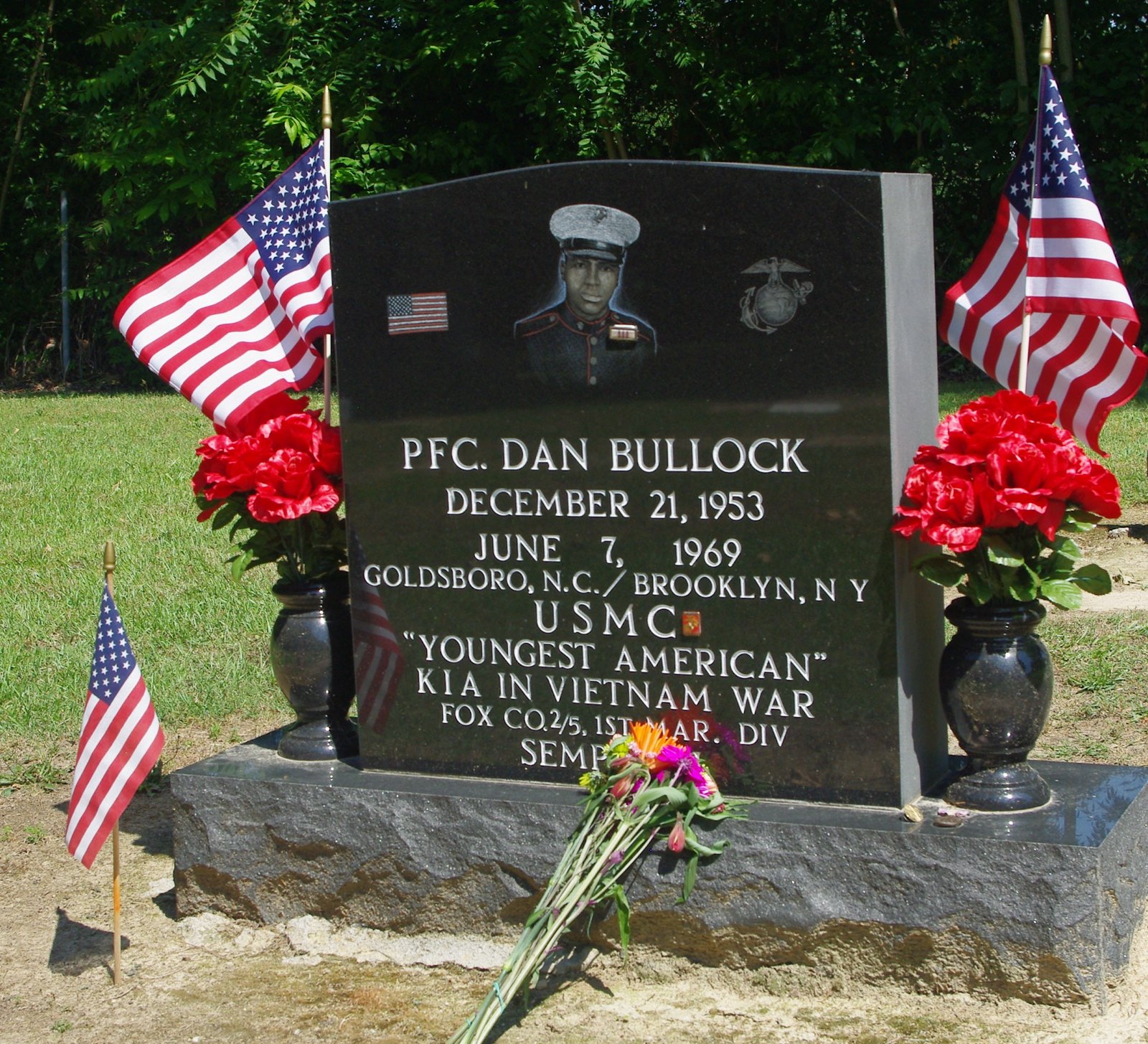The image is a color photograph centered on the gravestone of PFC Dan Bullock, prominently placed in a well-maintained grassy cemetery with lush green trees in the background. The gravestone features a portrait of PFC Dan Bullock, an African-American military serviceman dressed in a white military cap and dark blue uniform. To the left of his image is a small American flag emblem, and to the right is a small Marines emblem. The inscription beneath reads: "PFC Dan Bullock, December 21, 1953 - June 7, 1969, Goldsboro, North Carolina / Brooklyn, New York, USMC, 'youngest American KIA in Vietnam War', Fox CO. 2/5, 1st MAR. DIV". The lower part of the inscription is partially obscured but includes "SEMP". Flanking the gravestone are two black vases filled with vibrant red flowers. Additional details include three American flags: one on either side of the gravestone and one small flag planted in the soil in front. A small bouquet of pink and orange wildflowers lies at the base of the gravestone, adding a touch of color and memorial significance. The overall scene conveys respect and remembrance in a serene, green park-like setting.